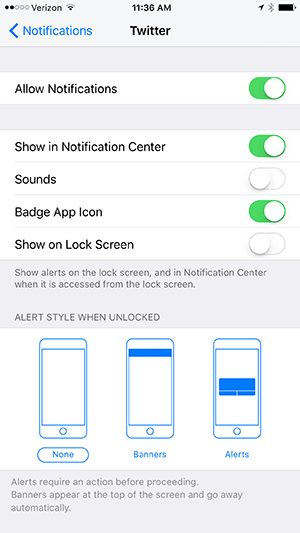In the detailed image caption user needs to clean up and elaborate on the voice description of settings sections: 

The image showcases the iPhone's system settings, specifically focusing on notification settings for the Twitter app. Within the main settings menu, the user has navigated to "Notifications" and selected the Twitter app. In the Twitter notification settings, several options are visible:

1. **Allow Notifications**: Enabled, allowing Twitter notifications.
   
2. **Notification Center**: Enabled, permitting notifications to appear in the Notification Center.

3. **Sounds**: Disabled, meaning no sound will play for incoming Twitter notifications.

4. **Badge App Icon**: Enabled, showing a small red circle with the number of unread notifications on the Twitter app icon.

5. **Lock Screen Notifications**: Disabled, preventing notifications from appearing on the lock screen.

6. **Notification Styles When Unlocked**: Offers the user three choices:
   - **None**: No notifications are displayed.
   - **Banners**: Temporary notifications that appear at the top of the screen and disappear automatically.
   - **Alerts**: Persistent notifications requiring user action before proceeding.

These settings allow the user to control how and when they receive Twitter notifications, offering a customizable experience for managing app alerts. Similar steps can be followed to configure notifications for each app on the iPhone.